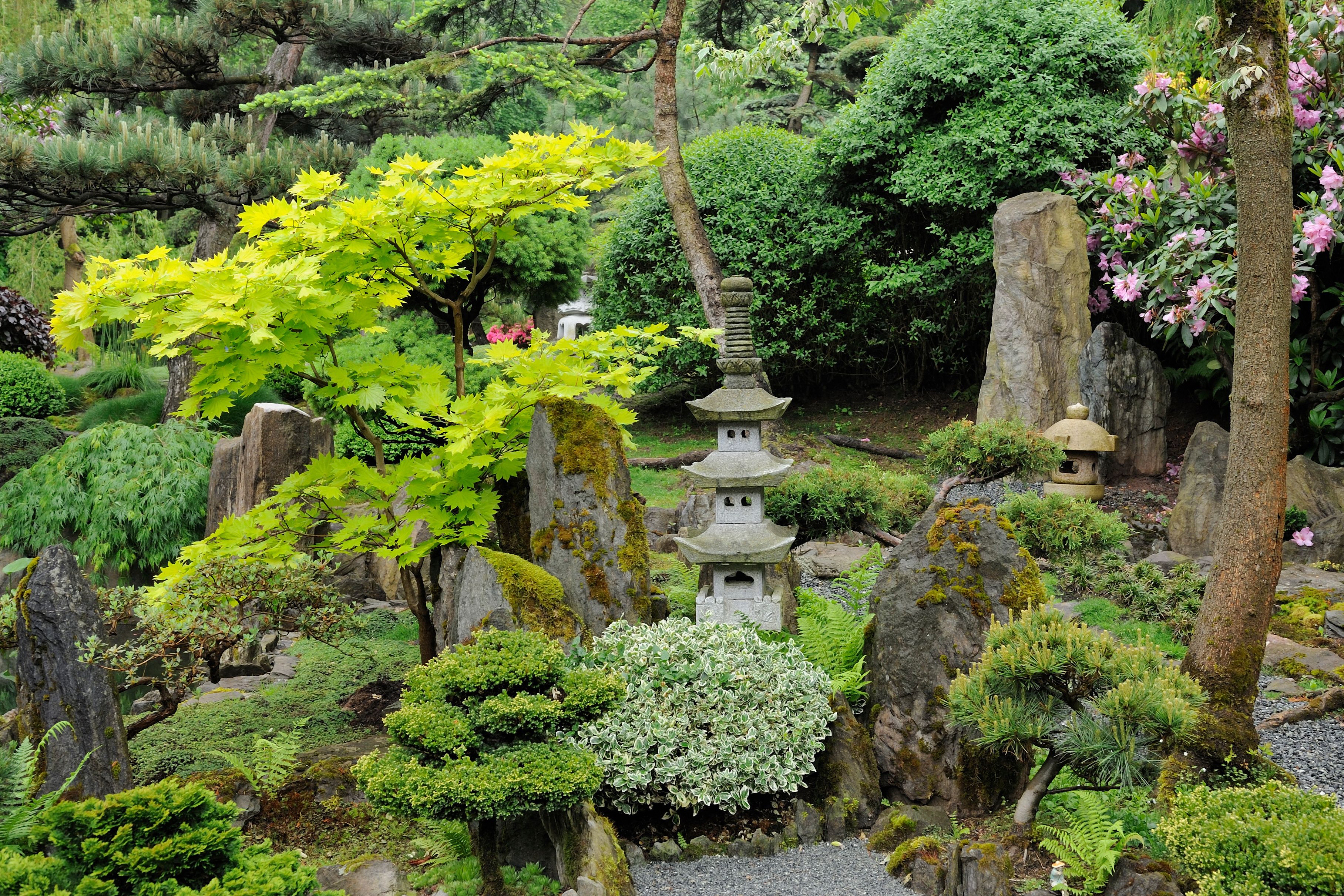The photograph captures an enchanting oriental garden, likely set in China, featuring a diverse range of plants, trees, and distinctive stone structures. The centerpiece is a multi-tiered, tall stone tower resembling a small Asian building. Surrounding this structure are different types of shrubs and trees, including a notably pretty pink bush tree in the far right corner. Moss-covered rocks can be seen in the center and to the left, adding to the garden’s natural, aged appearance. Walkways meander through the garden, inviting a tranquil stroll. Smaller ornamental buildings, reminiscent of miniature houses or birdhouses, are scattered throughout the scene, enhancing its cultural ambiance. The garden is lush with flora of various shades of green—from light and dark to sagey hues. The background features denser, larger trees, creating a lush and immersive environment. No people are visible in the photograph, emphasizing the serene and untouched beauty of this picturesque setting.